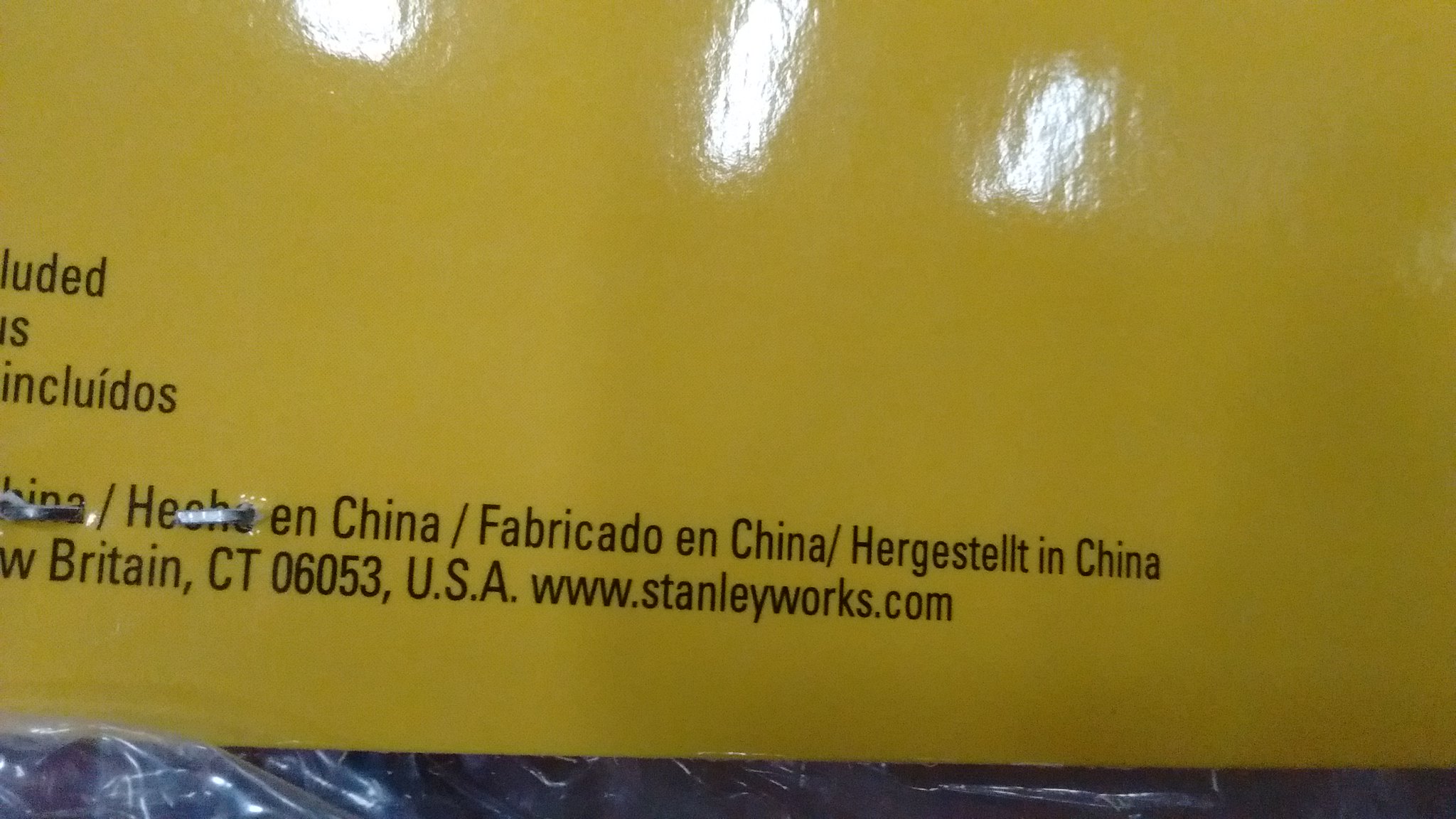The image depicts a polished, reflective yellow surface that prominently features various textual elements. In the top left corner, there are three white, shiny reflections. Below the reflections, the text reads "LUDED" followed by an "S" underneath it. Further down, it says "INCLUIDOS." Below this, the text continues with "HECHO EN CHINA / FABRICADO EN CHINA / HERGESTELLT IN CHINA." Additionally, there is a line that reads "BRITAIN, CTO 6053, U.S.A." Finally, at the bottom, the website "www.stanleyworks.com" is listed.